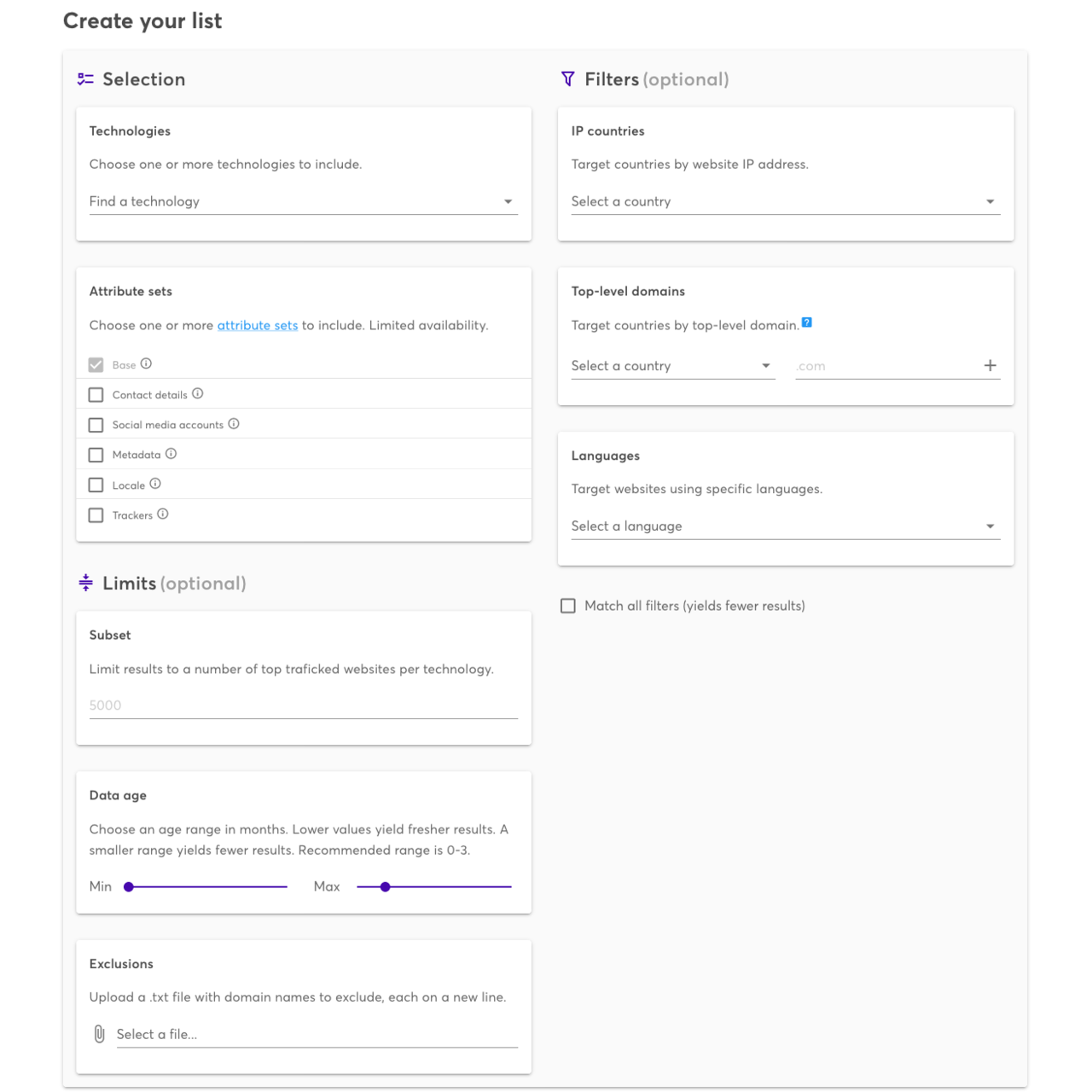The image depicts a webpage interface dedicated to the creation of a customized technology list. The header of the page prominently displays the title "Create Your List." The subsequent sections are outlined as follows:

### Selection:
**Technologies:** Users can choose one or more technologies to include in their list. The interface provides a search bar labeled "Find a Technology."

**Attribute Sets:** Users can select one or more attribute sets to include, such as 
- Base 
- Contact Details
- Social Media Accounts
- Metadata
- Locale
- Trackers

### Limits (Optional):
- **Subset:** Users can limit results to a specified number of top-trafficked websites per technology.
- **Data Age:** This section allows users to choose an age range in months for the data. Lower values yield fresher results, while a smaller range yields fewer results. The recommended range is 0 to 3 months. Users can set minimum and maximum values for this range.

### Exclusions:
Users can upload a TXT file containing domain names to be excluded from the list. Each domain name should be on a new line. A "Select a File" button is provided for uploads.

### Filters (Optional):
- **IP Countries:** Users can target countries by their website IP address, with an option to select a specific country.
- **Top-Level Domains:** Users can target countries by their top-level domain, with a dropdown menu to select a country.
- **Languages:** Users can target websites based on specific languages, with an option to select a language.

There is also an unchecked box that reads "Match All Filters," which, when selected, yields fewer results.

Overall, the web page provides a detailed and user-friendly interface for creating a customized list of technologies and attributes, complete with various filters and exclusion options to refine the search results.